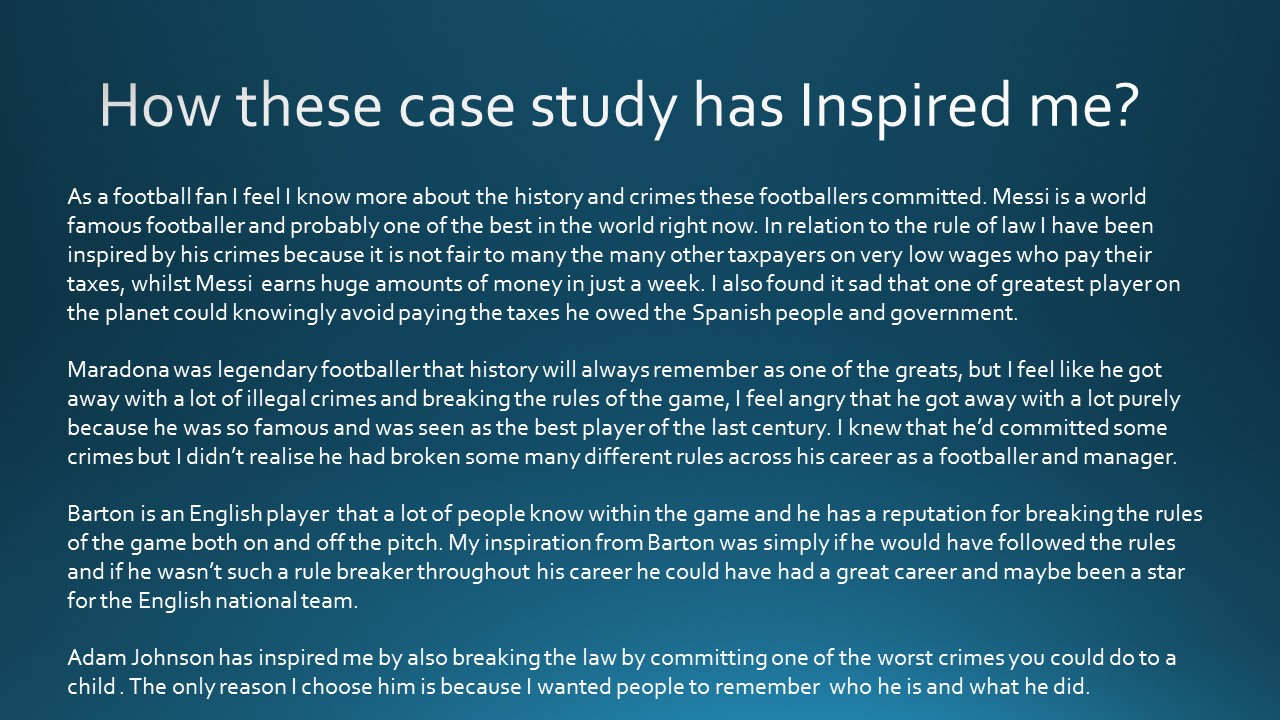The image depicts a slide displayed on a computer screen with a dark blue background and white text. The title at the top reads, "How These Case Studies Have Inspired Me." Underneath, in smaller writing, it states, "As a football fan, I feel I know more about the history and crimes these footballers committed." The slide discusses several well-known footballers and their legal issues.

It first highlights Messi, described as a world-famous footballer and one of the best in the world. The text expresses disillusionment with Messi for evading taxes, despite his immense earnings, which is seen as unfair to low-wage taxpayers who diligently pay their dues. There's a sense of sadness and disappointment that such a celebrated player would avoid his financial obligations to the Spanish people and government.

Next, Maradona is mentioned, remembered as a legendary footballer but criticized for evading legal consequences due to his fame. The narrator feels that his numerous infractions on and off the field were overlooked because of his status as one of the greatest players of the last century.

Barton, an English player known for his rule-breaking behavior, is also discussed. The text suggests that Barton's career could have been more illustrious if he had adhered to the rules, implying that his penchant for misconduct hindered his potential as a star for the England national team.

Finally, the slide mentions Adam Johnson, condemning him for committing severe crimes against a child. The narrator includes Johnson to ensure that people remember his actions and the severity of his offenses.

Overall, the slide conveys a deep sense of disappointment and reflection on how these footballers' crimes have influenced the narrator's perception of justice and fairness within the sport.